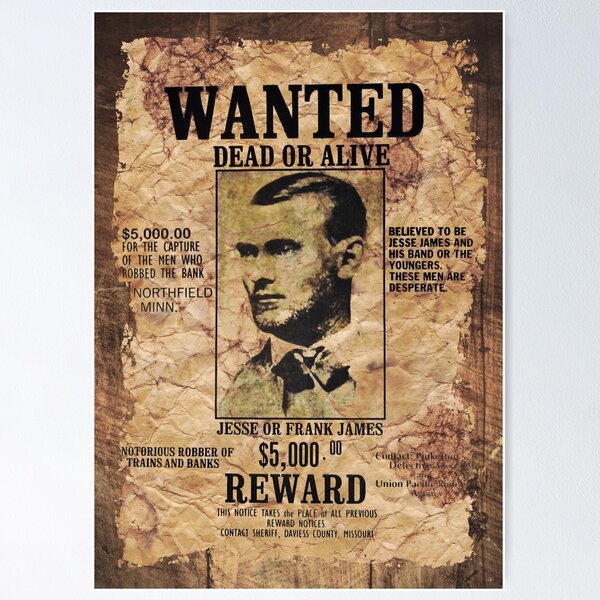This image is a highly detailed and weathered "Wanted" poster featuring notorious outlaws. The crumpled, tattered paper has a rustic look against a dark wood background. Across the top, in large black letters, the poster reads "WANTED," followed by "DEAD OR ALIVE" in smaller all-capital black letters. Below, it identifies "JESSE OR FRANK JAMES" with a "$5,000 REWARD." The poster describes the individuals as notorious robbers of trains and banks, specifically mentioning the robbery of a bank in Northfield, Minnesota. Beside the black-and-white profile photo of a man with combed-back dark hair and scruffy facial hair, it notes that $5,000 is offered for their capture. The text also indicates that these men are believed to be part of Jesse James' band or the Younger gang and are considered desperate. This notice supersedes all previous reward notices, directing anyone with information to contact Sheriff Davies County, Missouri.